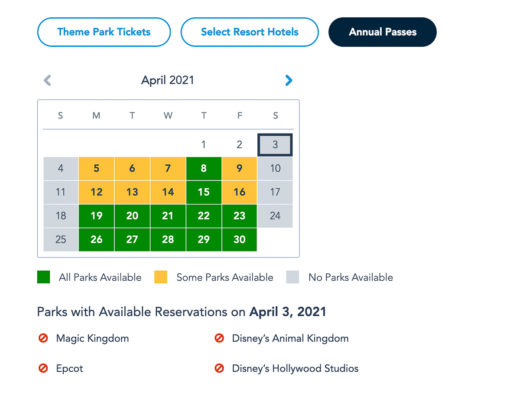Here is a cleaned-up and detailed caption:

"Set against a crisp white background, this image features a screenshot brimming with detailed information. At the top left corner, three distinct buttons are aligned horizontally: the first button, white with blue text, reads 'Theme Park Tickets'; to its right, a button outlined in blue with blue text reads 'Select Resort Hotels'; the third button, black with white text, reads 'Annual Passes'. Directly below these buttons is an image of a calendar displaying the month of April 2021 in subdued gray text. Notably, the date April 3rd is highlighted with a black outline and grayed out, indicating unavailability. Beneath the calendar lies a legend explaining the color codes: green signifies that all parks are available, yellow indicates that some parks are available, and gray denotes that no parks are available. Further below, bold gray text declares, 'Parks with available reservations on April 3rd, 2021,' emphasizing the date's importance. The structured layout and use of colors provide a clear and informative visual arrangement."